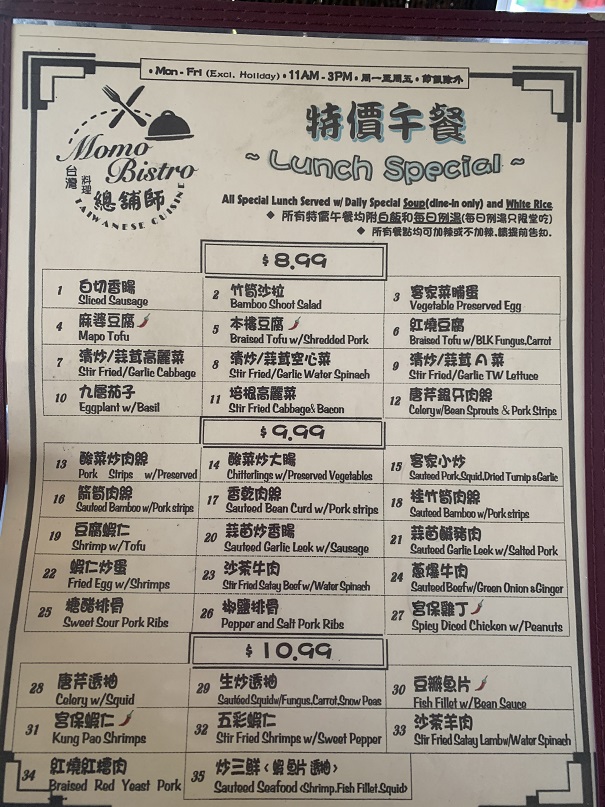This image depicts a detailed view of a laminated menu resting on a table. The menu features a thin border that frames a white laminated sheet. A prominent black border with thickened corners further enhances the design, adding a touch of elegance with delicate white etchings in the corners.

At the center of the menu, a white rectangle states, in black lettering, "Monday through Friday, excluding holidays, 11 a.m. to 3 p.m." This section is headed by the word "Monday" and is accompanied by Chinese characters.

A circle motif adorns the upper portion of the menu. Within this circle, at the top, crossed knife and fork icons are present, with the knife pointing to the upper right and the fork to the upper left. Just beneath this, the name “Momo Bistro” is displayed in bold black lettering, followed by Chinese characters. At the bottom of the circle, the label “Taiwanese cuisine” is inscribed.

To the right of the circle, a small bell, reminiscent of those found in shops for ringing, is depicted. Adjacent to this, the text "Lunch Special" is prominently displayed in large lettering. Below this heading, the main body of the menu lists various dishes along with their prices, described primarily in Asian script, with some English translations provided underneath.